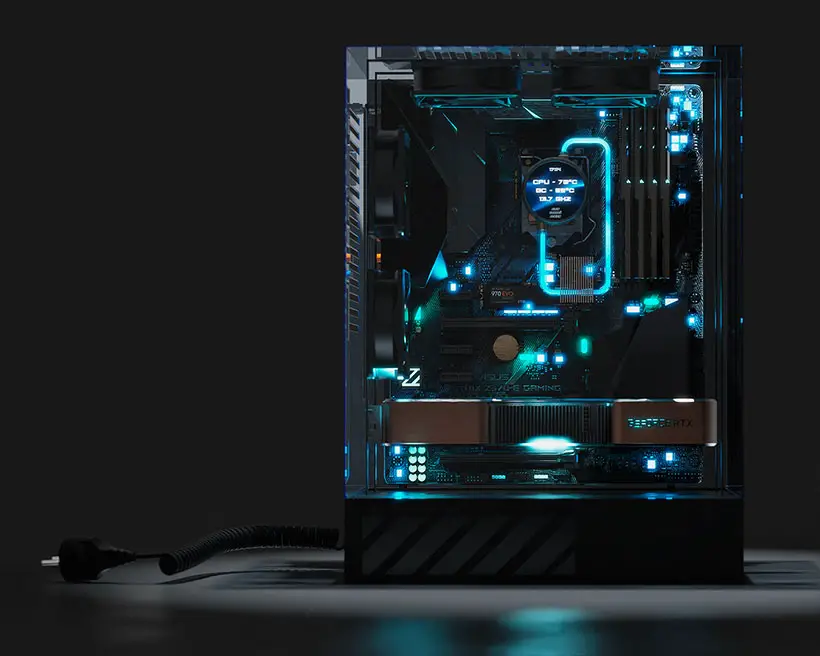The image depicts a custom-built, rectangular, crystal-clear PC tower placed on a dark-colored surface against a black wall. The sides of the case are completely removed, providing a full view of the internal components. Dominating the center of the case is a notable circular blue-lit display with a rectangular blue light-up area connected to it. This display prominently features the label "CPU-78C" with additional, less-readable numbers and letters underneath suggesting specifications such as "SC-55C." Inside the case, blue and green lights illuminate various components, including the cooling lines and fans, adding a vibrant glow to the internal hardware. Some parts bear the branding "ASUS" and include references to gaming. A coiled wire extends out from the left bottom corner of the case, and overall, the internal setup includes meticulously placed and sometimes glowing screws, wires, and other hardware components.